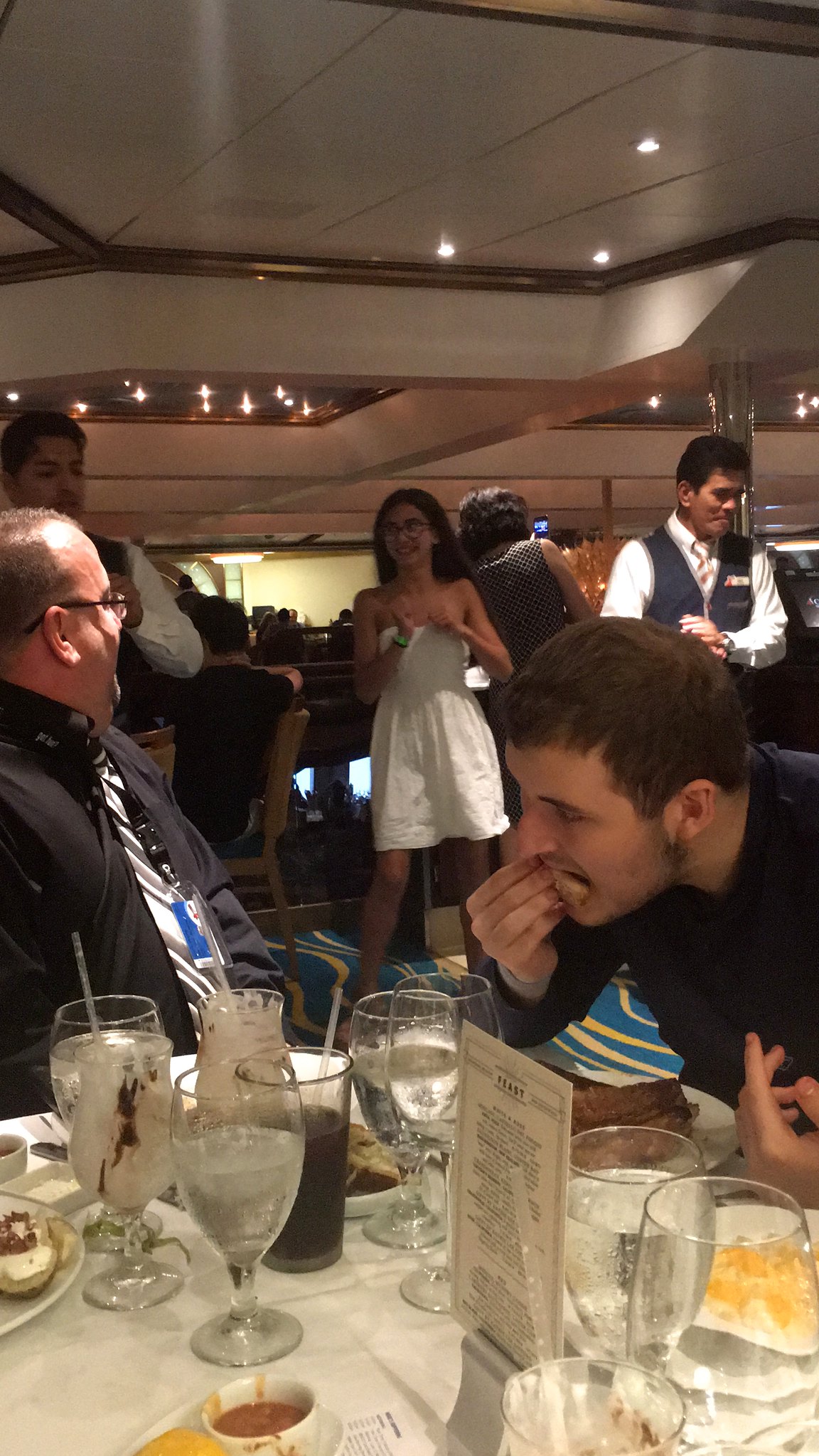The image captures a lively indoor event, possibly at a hotel or convention center, set in portrait mode. The scene centers around a table in the foreground, draped with a white tablecloth and cluttered with numerous water glasses, soda glasses with straws, and a white ceramic bowl that may contain some sauce next to what appears to be bread.

To the right, a man dressed in a dark black shirt is caught mid-bite, leaning over the table as he eats. Beside him, another man, also in a dark shirt and accented with a tie that features black and gray tones with hints of blue—or possibly a name tag—observes the scene. This man has light brown, balding hair and wears black glasses.

At the center, a woman in a short, white strapless dress with long black hair flowing behind her shoulders and wearing glasses stands out. She appears to be dancing or holding her hands up in a joyful gesture. In the background is a waiter or bartender in a black vest, white button-down shirt, and a name tag, adding a touch of formality to the setting.

The upper portion of the image reveals a ceiling transitioning from white to a coppery hue, dotted with lights, while the background is marked by a wave-patterned blue carpet interwoven with gold. Additional tables, a woman in a shoulderless jumpsuit smiling, and more diners contribute layers of activity and festivity to the scene. The overall ambiance suggests the lively conclusion of a meal, surrounded by happy attendees and attentive service staff.